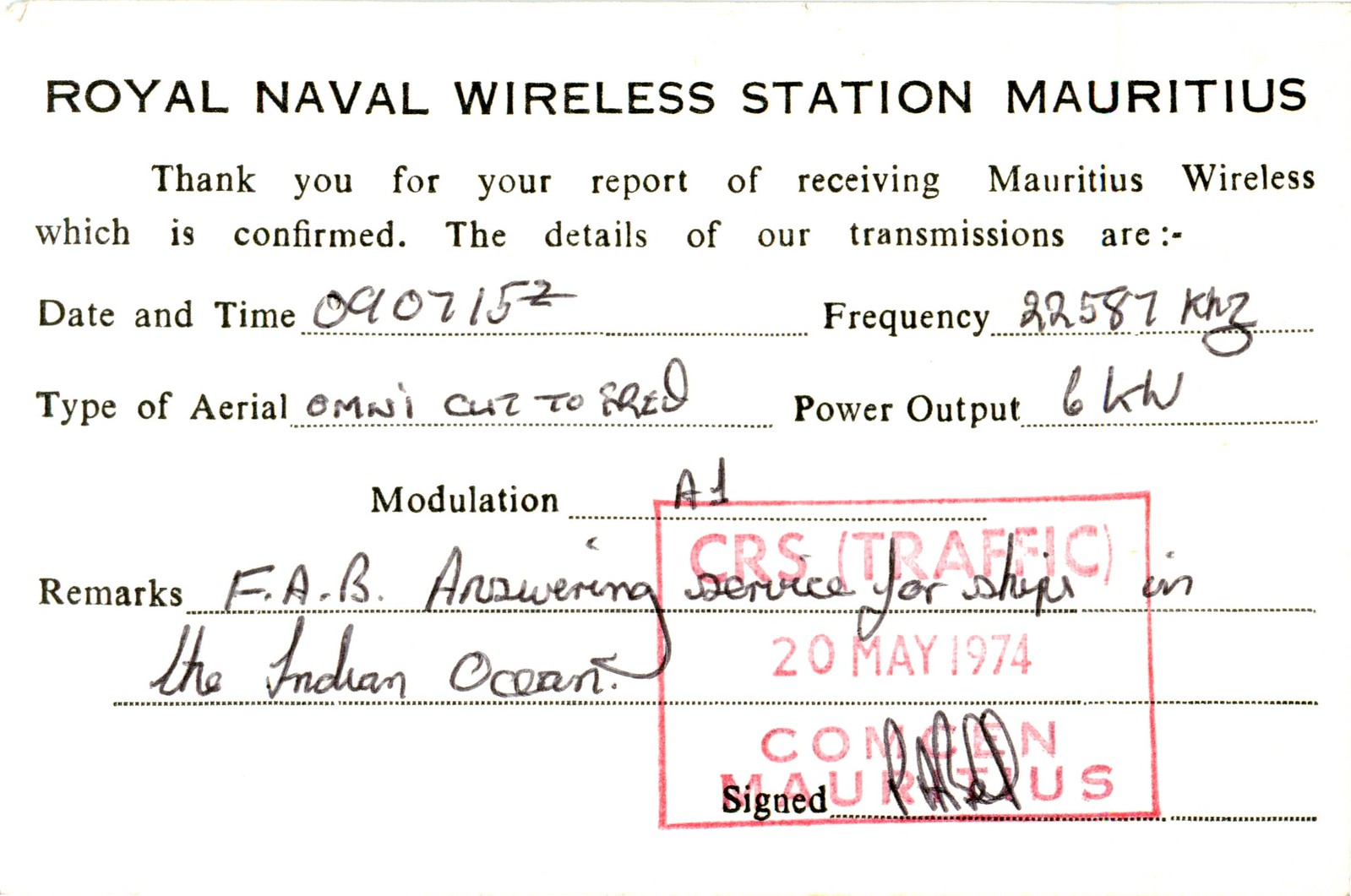This image features a horizontally oriented card that occupies nearly the entire frame. Predominantly in black, white, and red, it bears the header "Royal Naval Wireless Station, Mauritius" in bold, all-caps black lettering. Below this, in smaller black type, is the message: "Thank you for your report of receiving Mauritius Wireless, which is confirmed." The transmission details are provided next: "Date and time: 0907152," "Frequency: 22587kHz," "Type of aerial: Omnicuz2red," "Power output: 6KW," "Modulation: A1," "Remarks: FAB, answering service for ships in the Indian Ocean." Additionally, a red stamp marked "CRS traffic, 20 May 1974, Mauritius" and a handwritten signature are also visible, emphasizing its authenticity and official nature. The card appears to serve as a formal confirmation receipt from a naval wireless station potentially related to maritime communication.